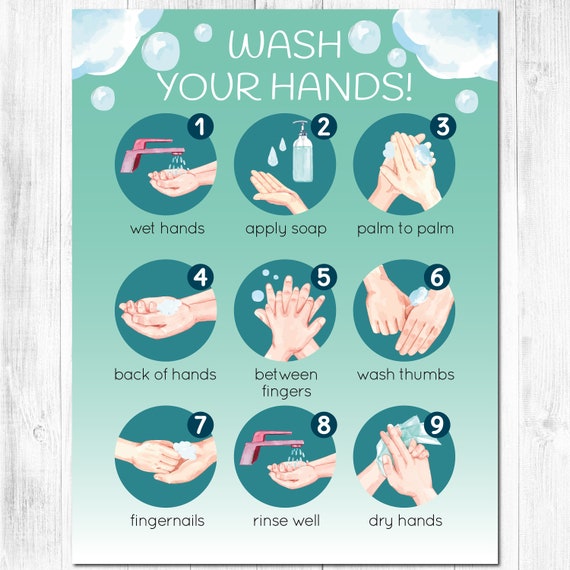The infographic, titled "Wash Your Hands," serves as a detailed instructional guide on proper hand-washing techniques, set against a predominantly green background that transitions to white at the bottom, with soap bubbles adorning the top corners. The process is broken down into nine clearly numbered steps, each depicted within a blue circle. Below each circle is a concise instruction in white text:

1. A hand under running water with the caption "Wet hands."
2. Soap being applied to the hands with "Apply soap."
3. Two hands rubbing together labeled "Palm to palm," illustrating the initial soap lathering.
4. Scrubbing the back of the hands, captioned "Back of hands," to ensure thorough cleaning.
5. Washing between the fingers, denoted as "Between fingers."
6. Cleaning the thumbs, under the instruction "Wash thumbs."
7. Scrubbing the fingernails, labeled "Fingernails."
8. Rinsing the hands under a faucet with "Rinse well."
9. Drying the hands with paper towels, captioned "Dry hands."

This comprehensive visual aid effectively emphasizes the sequential steps necessary for proper hand hygiene, utilizing clear illustrations and descriptive captions for each stage.